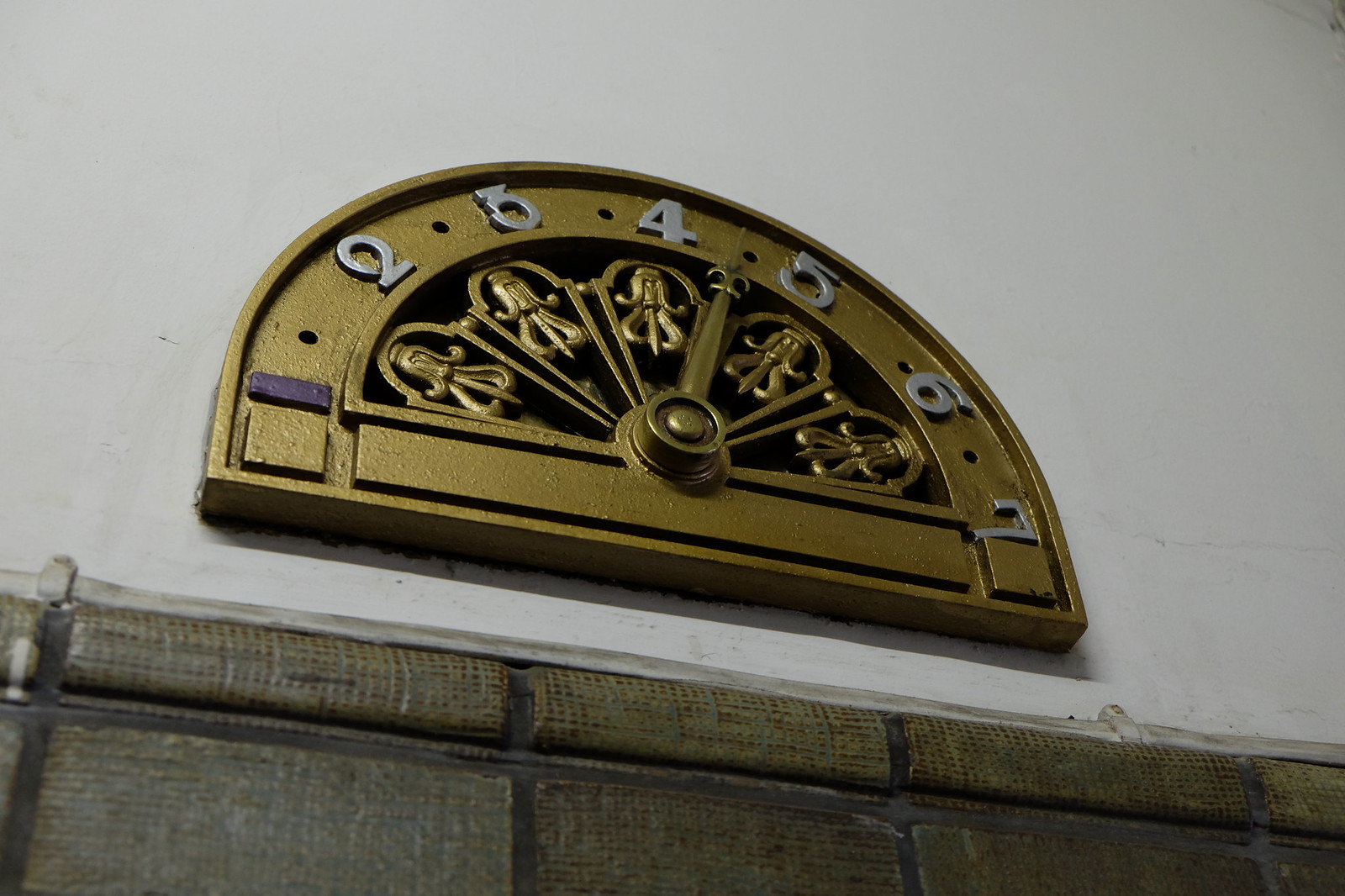This photograph captures an antique elevator indicator, characterized by its semi-circular gold design. The ornate half-circle features numbers one through seven, arranged elegantly along its arch, with the number four prominently positioned at the apex. A decorative gold arrow points precisely between the numbers four and five, suggesting the elevator's current position. The design evokes the appearance of a clock face, enhancing its vintage charm and functional elegance. The background is a stark white wall, which contrasts sharply with the blackish-gray structure below, hinting at the elevator's aged, yet sturdy build. The close-up perspective brings the intricate details of the indicator into sharp focus, making it the centerpiece of the image.